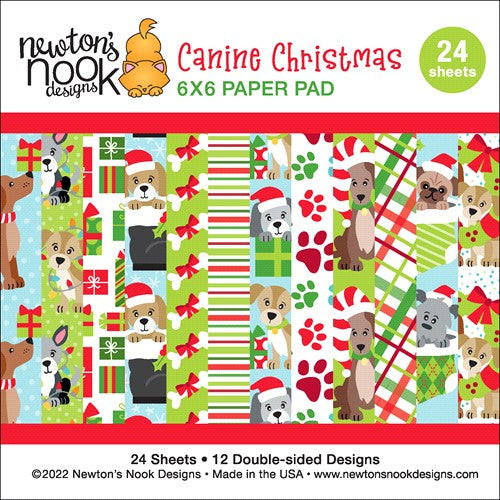The front of the packaging for a 6x6-inch paper pad features a thicker white border at the top, highlighting key details in black lettering on the top left that read "Newton's Nook Designs." Adorning this section is a playful illustration of a little orange or yellow cat stretching. Below the brand name, prominent red letters spell out "Canine Christmas," followed by "6x6 Paper Pad" in green text. 

A round green circle on the right side of the package states "24 Sheets" in white letters. The central area showcases a charming cartoon design with various dog breeds, including a recognizable pug among the mix, though the rest are less distinguishable. The overall theme is festive, featuring elements like red and green stripes, orange paw prints, red bows, and white bones, all capturing the Christmas spirit.

Additional information at the bottom notes that the pad consists of "24 sheets, 12 double-sided designs," and is marked with "2022 Newton's Nook Designs," emphasizing that the product is "Made in the USA."